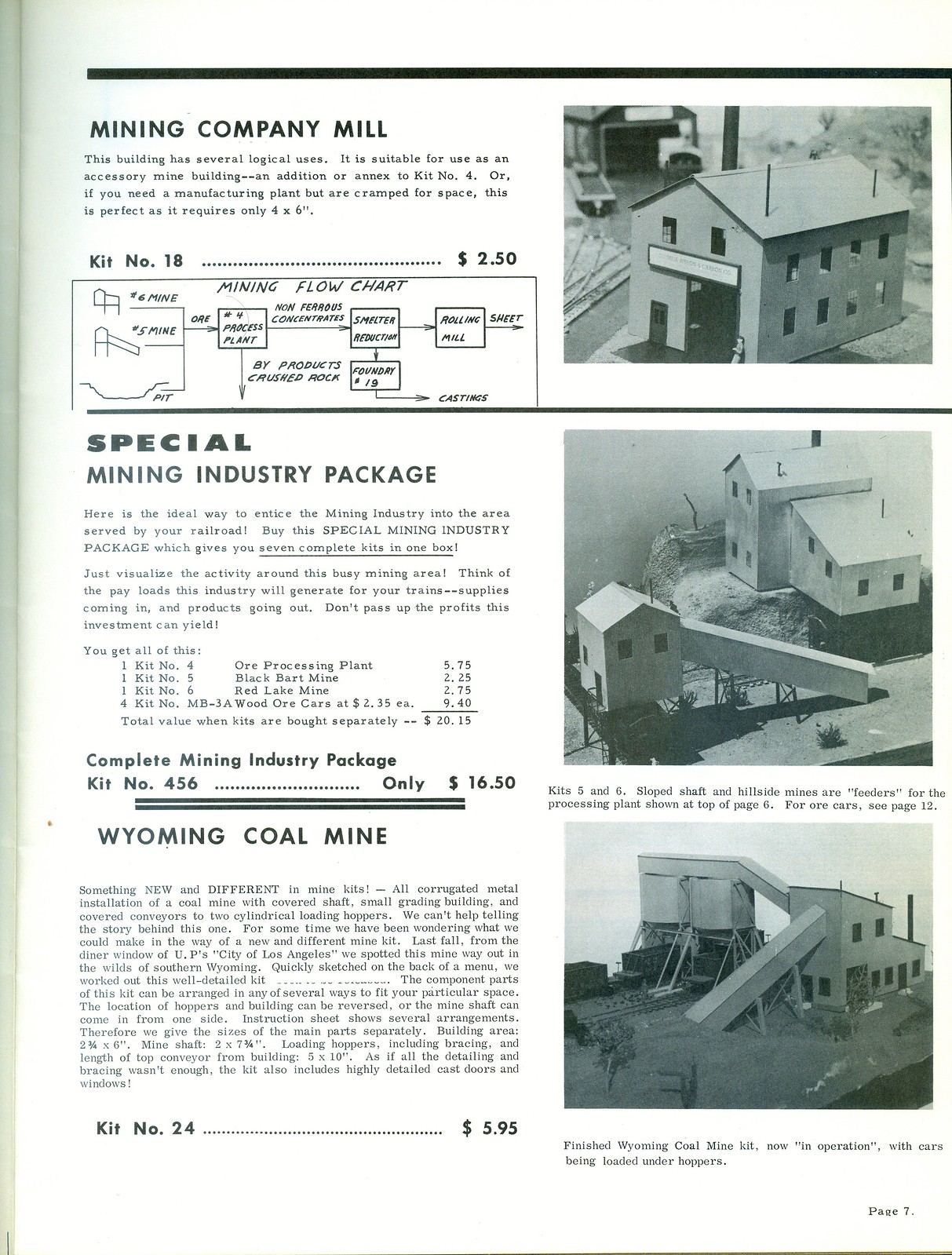The image shows an advertisement from an older magazine, likely for miniature building kits suited for model railroads or dioramas. The advertisement spans one page, which is upright and taller than it is wide, with a visible fold on the left edge, indicating it's the right-hand page of an open book.

The page is divided into three distinct horizontal sections, each promoting a different building kit:

1. **Mining Company Mill**
   - **Description:** This kit, labeled as kit number 18, is described as versatile for use as an accessory mine building or a compact manufacturing plant, requiring only a 4x6 inch space.
   - **Price:** $2.50
   - **Image:** A simple, two-story rectangular building with a triangular roof is displayed, alongside a mining flowchart diagram for context.

2. **Special Mining Industry Package**
   - **Description:** Titled as the Complete Mining Industry Package (kit number 456), this set is detailed extensively, explaining that it consists of multiple structures, including three buildings, with one featuring a chute. The special package is capable of integrating sloped shaft and hillside mines, designed as feeders for a processing plant.
   - **Price:** $16.50
   - **Image:** A collection of three interconnected buildings, including apparatuses like chutes for ore transfer, suitable for a fully operational mining setup.

3. **Wyoming Coal Mine**
   - **Description:** This kit, marketed as kit number 24, includes a detailed two-story building with dual chutes—one extending down to the ground and another running over grain silos toward railway cars. The description emphasizes its utility for loading cars under hoppers efficiently.
   - **Price:** $5.95
   - **Image:** Displays the connected box-like buildings, highlighting the operational coal mine setup loading railway cars.

The entire advertisement is rendered in black and white, reinforcing its vintage nature, and it effectively provides a glimpse into the intricate detail and artistry involved in creating realistic miniature mining scenes.